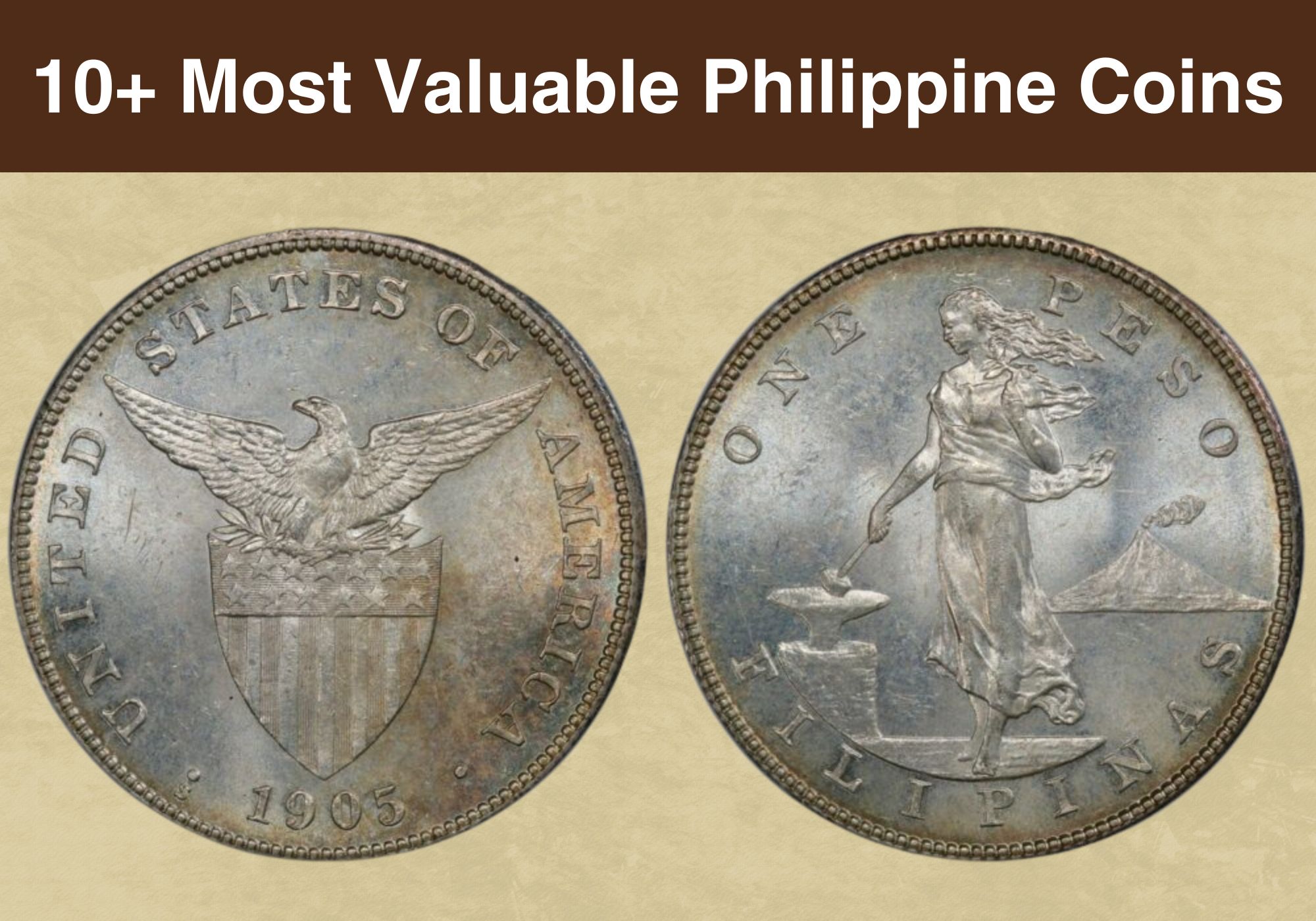The image showcases a photograph of two antique collectible coins against a solid beige background. At the top, a brown horizontal strip with white text reads, "10+ Most Valuable Philippine Coins." On the left, a coin dated 1905 features the inscription "United States of America" around its border, with a central design displaying a shield topped by an eagle. The coin on the right, labeled "One Peso," displays a female figure with long flowing hair, dressed in a Grecian robe, standing on a platform and striking an anvil. The inscription "Filipinas" is at the bottom, and in the distance, there is a depiction of a volcano. The coins are silver but appear weathered, adding to their antique charm. The image uses a photographic representationalism style with elements of realism and graphic design.